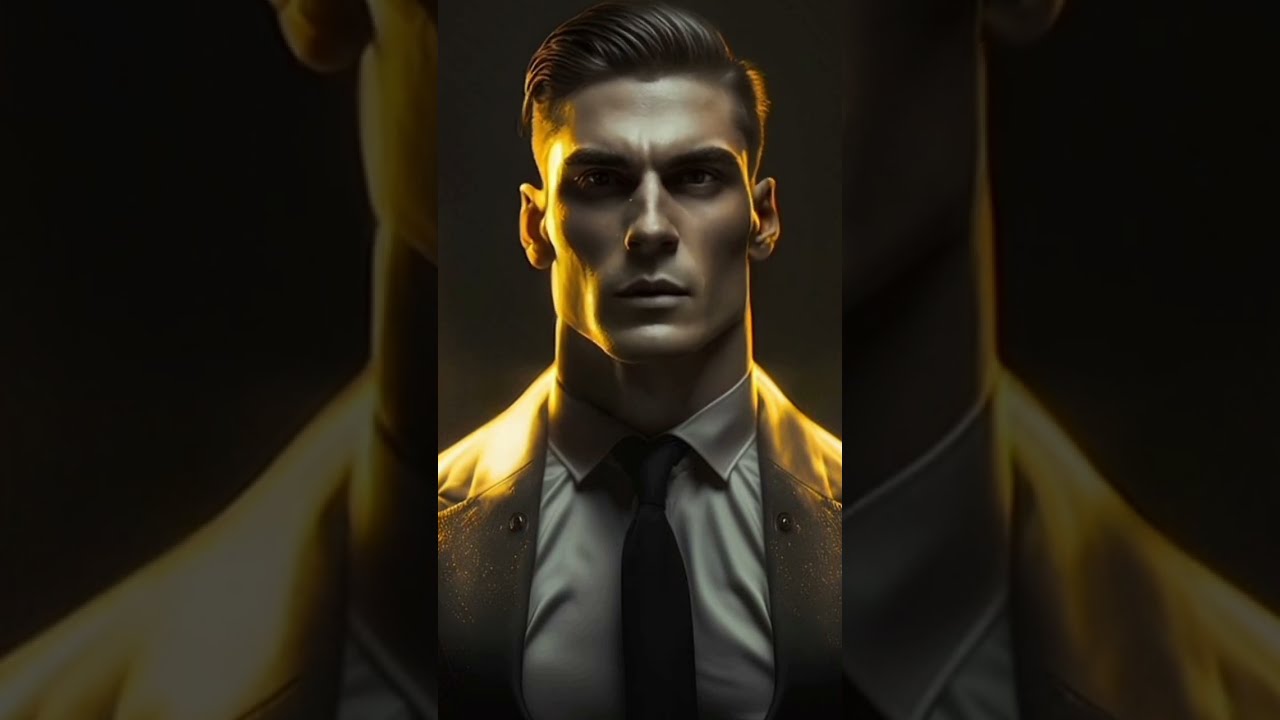This is an AI-generated image featuring a striking, animated portrait of a handsome young man. The image is divided into three vertical strips, with the central strip containing the sharp, clear portrait, while the strips on either side display zoomed-in, faded versions of the same portrait. The man has neatly coiffed brown hair, styled in a comb-over with short sides, and he sports a serious expression on his clean-shaven face. He wears a light brown blazer over a gray dress shirt and a black tie, with golden light illuminating the sides of his face and the top of his blazer. The background is slightly dark brown, enhancing the focus on the central portrait. The placement of the camera, slightly below his jawline, emphasizes his sharp jawline and fit physique.